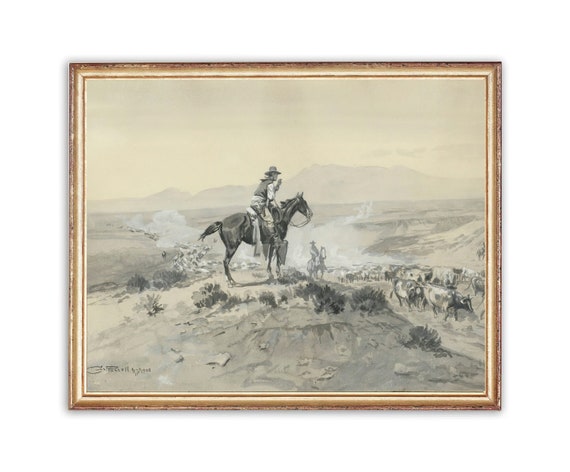The image depicts a detailed, hand-drawn sketch of a cowboy sitting atop a horse, framed in a ornate gold frame. The artwork, predominantly in shades of black, white, gray, and tan, captures the cowboy with a hat, vest, and white shirt, holding the reins as a blanket drapes over the horse's back, which is fully saddled. In the background, a range of barely visible, faint gray mountains stretch across the horizon under a dull sky. Rough hills and scrubby terrain populate the scene, with a few cattle or sheep positioned on the right-hand side. A second figure on horseback is subtly included in the distance, adding depth to the composition. The lower left part of the sketch contains some barely legible text, and scattered tumbleweeds accentuate the rugged landscape. Despite its monochromatic palette, the image exudes a rustic beauty and high-quality craftsmanship.